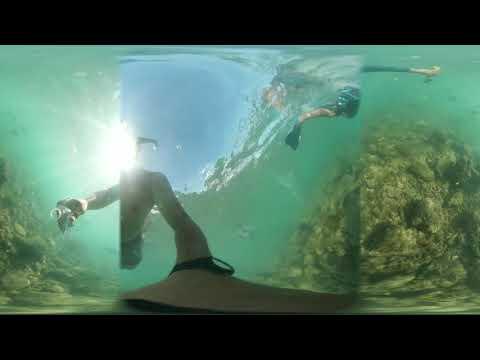The photograph showcases an underwater scene brimming with detail and vibrant life, captured perhaps during a scuba diving adventure. The bluish-green water displays varying shades due to the interplay of sunlight and underwater shadows. At the forefront, an arm extends from the left-center, nearly touching the bottom with a black watch visible on the wrist, belonging to a shirtless person in swimming trunks. Not far from this, another person's right hand appears, gripping a suction cup, emphasizing the multitude of activities or tasks happening underwater. Brownish-green rocks and large pieces of coral form the backdrop and foreground of the scene, with rocky outcrops contributing to the underwater terrain.

Amidst this aquatic environment, the top of the water surface gleams with daylight, showing hints of sky-blue above. To the top right of the picture, only a diver's foot paddles and an outstretched arm, wearing black trunks, are visible as they swim out of view. Adding depth to the scene, the background reveals a mix of clear and slightly murky water, suggesting varying distances and depths. A long black horizontal bar runs across the top and bottom of this panoramic 360-degree image, enhancing the immersive feel of the underwater adventure.